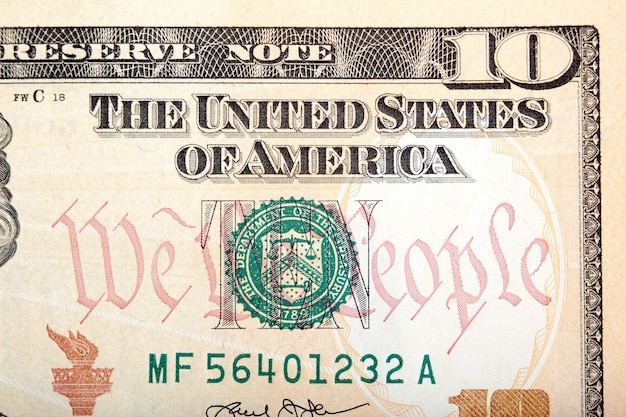This landscape-oriented photograph captures the upper right section of a U.S. $10 bill. In the top right corner, a bold "10" signifies the denomination. Directly beneath, the inscription "THE UNITED STATES OF AMERICA" is clearly visible in large black capital letters. Below that, the phrase "We the People" is elegantly scripted in a light, semi-transparent red, with a faint "10" superimposed in the background.

Overlaying part of the text is the green Department of the Treasury seal, making duplication difficult. The intricate black border frames the top of the bill with "RESERVE NOTE" detailed inside it. The serial number "MF56401232A" appears in a dark green hue near the center. To the left of the serial number is an orangish torch, reminiscent of the Statue of Liberty's torch.

Further down, a black cursive signature is present, and another "10" in an orangish-red color can be seen in the lower right corner. Though the photo does not show Alexander Hamilton's face, a hint of his hair is visible, indicating his presence on the left part of the bill. The overall paper color of the bill has a light brownish-gray tint, adding to its detailed design.